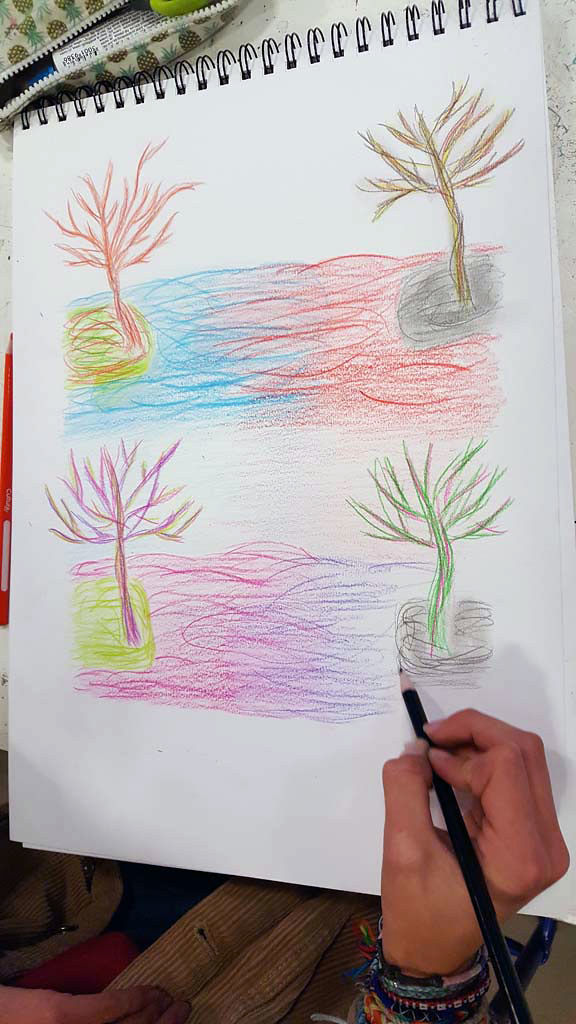This image appears to be a detailed colored pencil sketch on a plain white sheet of paper in a notebook with a black spiral binding at the top. The notebook's simple design contrasts with the vibrant colors and intricate details of the artwork. At the bottom of the sheet, a tan-skinned hand adorned with multiple bracelets firmly grips a black colored pencil. The sketch itself features two distinct scenes, both depicting a body of water with two small islands, each crowned by a single tree. Although the composition of both scenes is similar, the artist has used different colors for the water, islands, and trees, giving each image a unique feel despite their identical layouts.